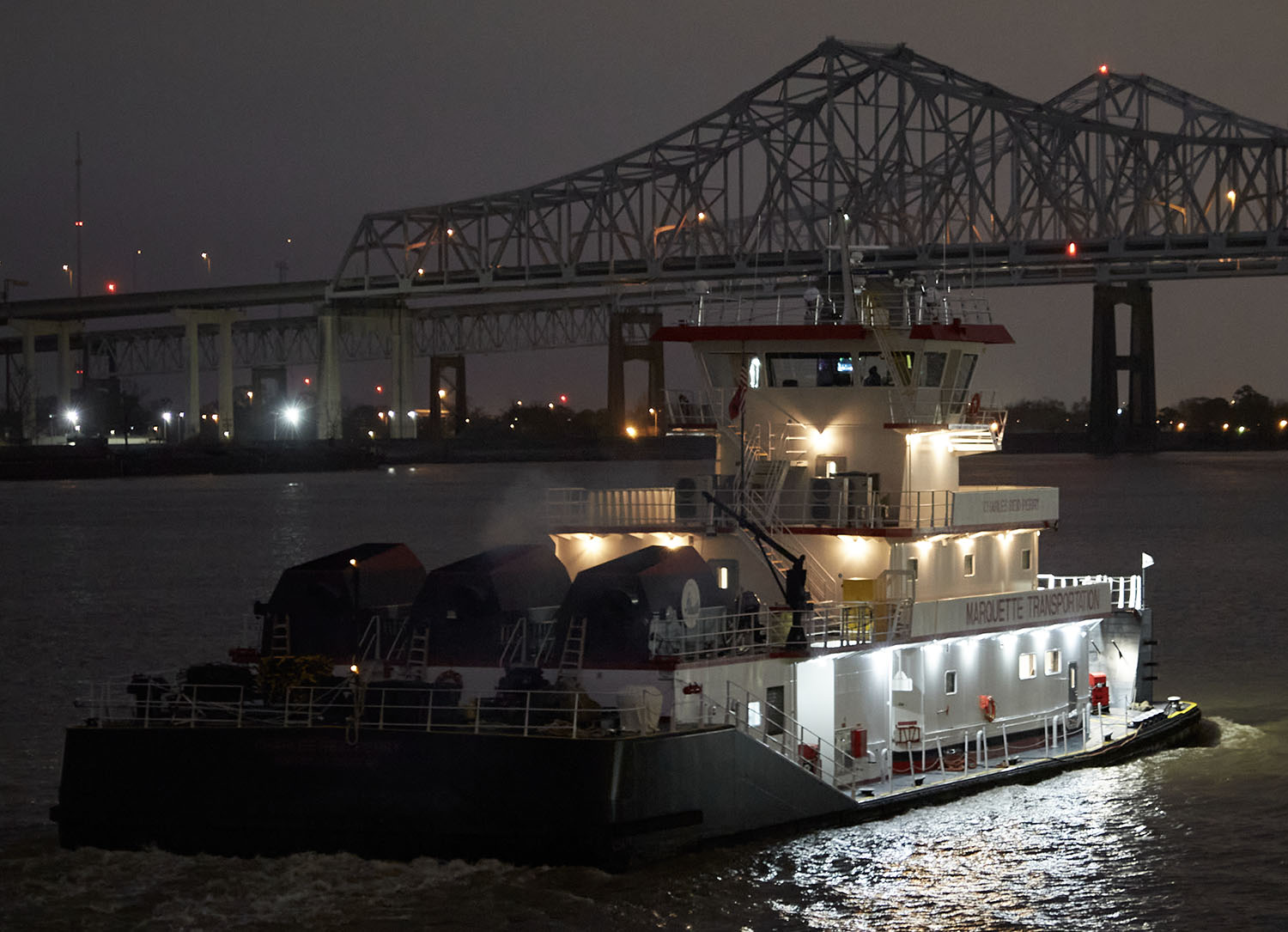This nighttime image captures a large, multi-level boat, marked “Marquette Transportation,” navigating a body of water beneath an imposing, illuminated bridge. The boat's lower section glows brightly through numerous windows, while the upper levels are bathed in a warm light emanating from smaller windows. The top-most level, which appears to be the control room enclosed in glass, silhouettes a man and displays faint screens. Encased in the dusky, overcast sky, the scene is layered with reflections and city lights scattered along the distant shoreline. The A-framed bridge rises dominantly above the boat with white scaffolding and sparse lights dotting its structure, adding to the urban ambiance. Despite the absence of visible traffic on the bridge, numerous minute lights indicate an adjacent, perhaps industrial, waterside vicinity, casting a serene yet bustling nocturnal atmosphere.